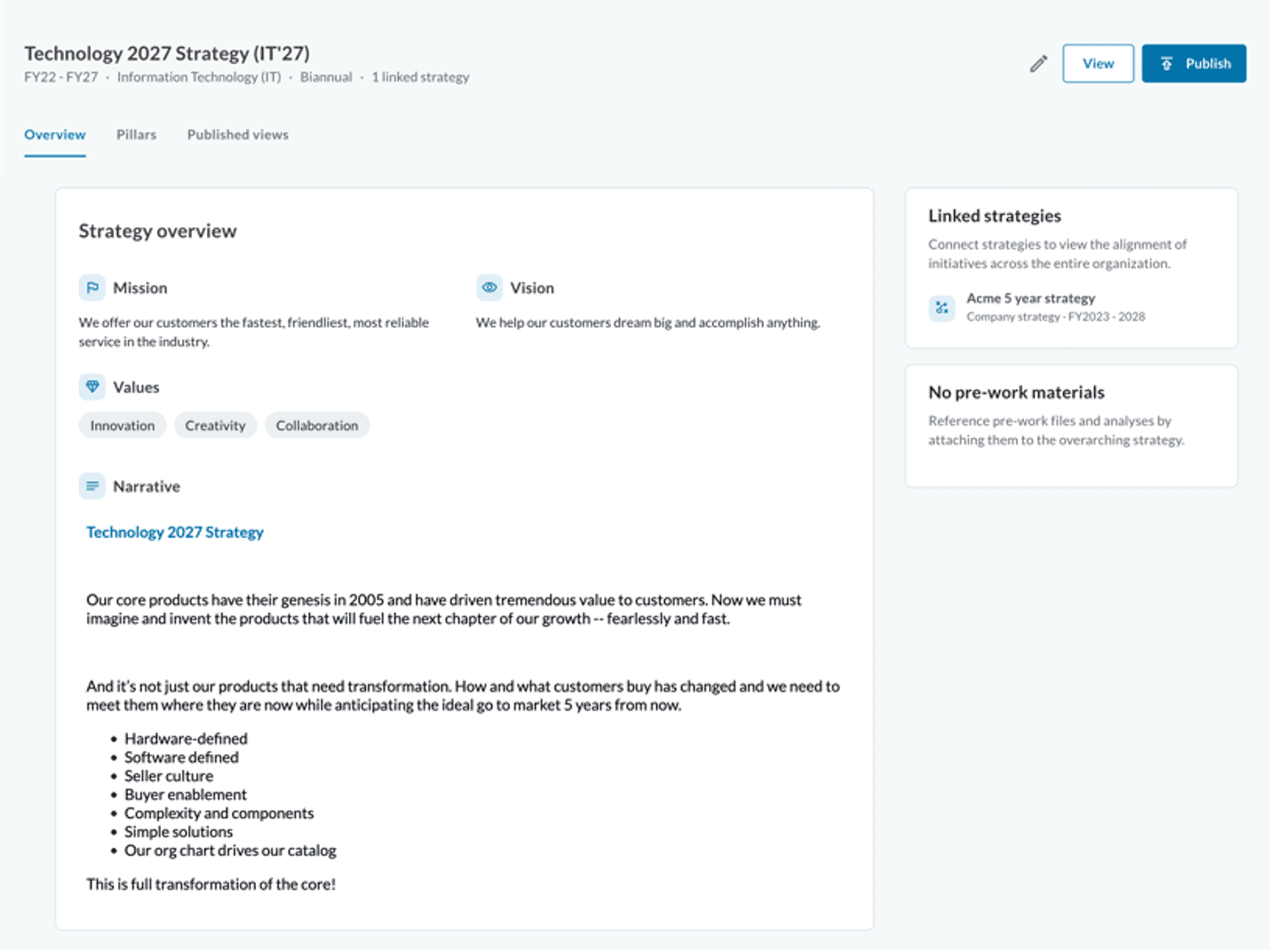### Detailed Strategy Overview for Technology 2027

This detailed strategy overview pertains to the "Technology 2027 Strategy" initiative by a company, highlighting its FY27 Information Technology (IT) biannual one-link strategy. 

At the top of the document, the title "Technology 2027 Strategy" is prominently displayed. Below this main header, the subheading includes "FY TT FY27 Information Technology IT Biannual One-Link Strategy" with additional navigation options such as Overview, Pillars, and Published Views. The active selection, Overview, is highlighted in blue, while the remaining options are in black.

On the right-hand side of the document, users have the options "View" and "Publish," which are presented in blue and white fonts. A pencil icon beneath these options is accompanied by another actionable item labeled "Link Strategies," designed to connect different strategies and view the alignment of initiatives across the entire organization. This includes the ACME Five-Year Strategy covering FY 2023 to 2028.

Centrally positioned, the document notes that there are no pre-work materials required. Below this, the core strategy is outlined, focusing on the Mission, Vision, Values, and Narrative:

- **Mission:** "We offer our customers the latest, friendliest, most reliable service in the industry."
- **Vision:** "To help customers dream big and accomplish anything through high user innovation, creativity, and collaboration."
- **Narrative:** "The Technology 2027 Strategy builds on our core products, initiated in 2005, which have delivered substantial value to our customers. As we look toward the future, we must conceive and develop products that will propel our next phase of growth, doing so with fearlessness and speed. Not only our products but also the ways in which our customers purchase them have evolved. We must meet customers where they are now while forecasting the ideal go-to-market strategy five years ahead. This entails transitioning from hardware-defined to software-defined solutions, fostering a seller culture, enabling buyers, simplifying complexity, and delivering streamlined solutions. Our organizational structure drives our comprehensive catalog, marking a full-scale transformation at the core."

Below this narrative, the document dissected elements such as hardware-defined and software-defined solutions, seller culture, buyer enablement, and the simplicity of complex components. The organization's overarching mission is to deliver clear and efficient solutions that drive their complete transformation agenda.

By capturing the scope of the Technology 2027 Strategy meticulously, the company aims to ensure clarity, alignment, and focused progress across all strategic initiatives over the next five years.